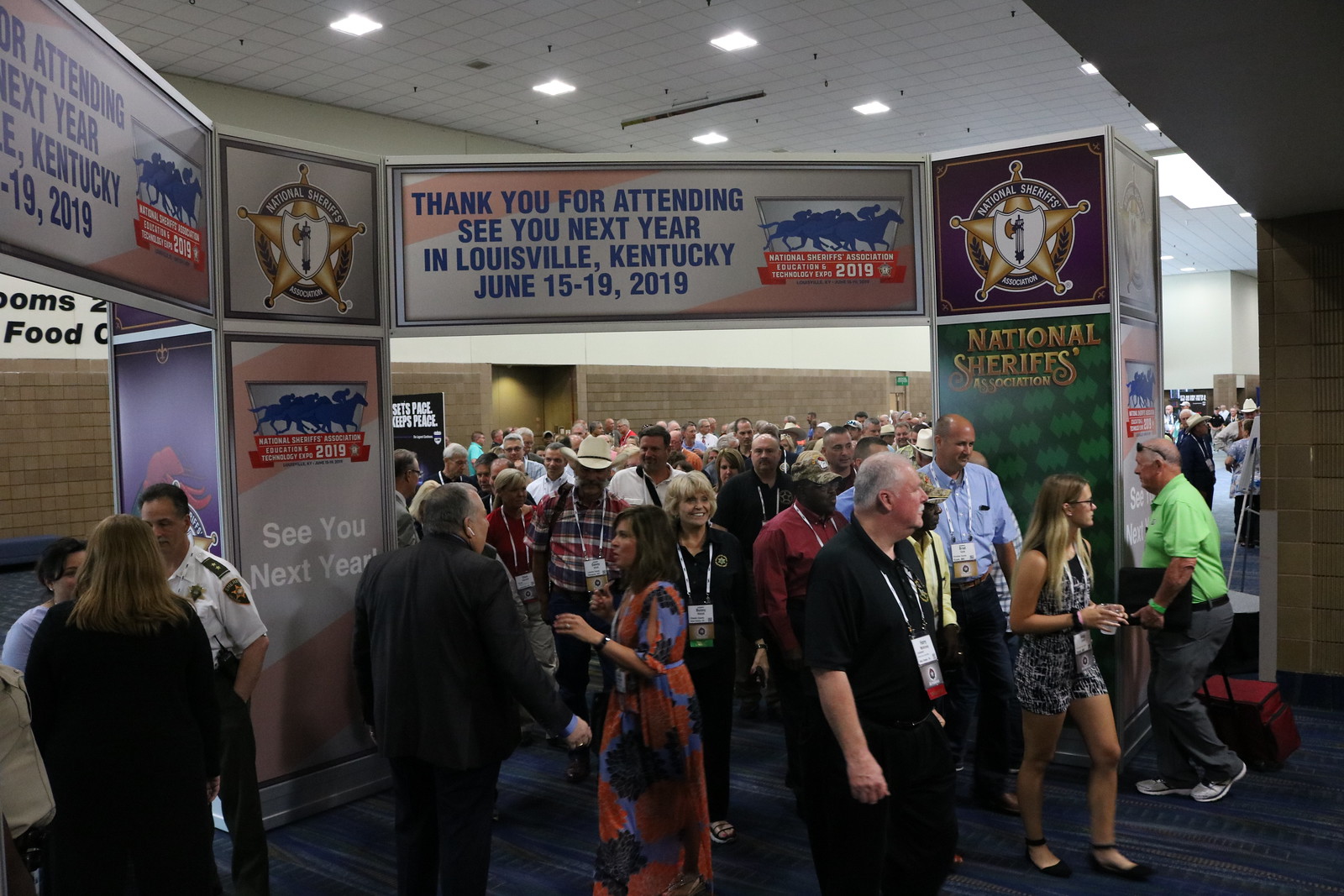In the image, the scene captures the exit of a large event, likely held at a convention center, given the setting and details. A crowd, predominantly composed of older white individuals, is streaming under an archway adorned with various banners and signs. The signage prominently displays messages such as "Thank you for attending. See you next year in Louisville, Kentucky, June 15th through 19th, 2019," alongside logos resembling sheriff's badges and slogans from the National Sheriff's Association. Many individuals in the crowd are wearing lanyards, indicating their participation in the event, with some sporting cowboy hats and dark clothes. Notably, an older, bald gentleman with gray hair is clearly visible, distinguished by a convention badge around his neck, and another man wearing a green shirt stands to the far right. A uniformed individual with a white shirt and a shield or badge on his arm is positioned to the far left. The crowd flows over blue carpeting and is captured against a backdrop featuring a brown tiled lower wall and a white upper wall, all under a ceiling with tiles and fluorescent lights. The overall mood suggests the conclusion of a sizable, organized event, with attendees making their way towards the exit.